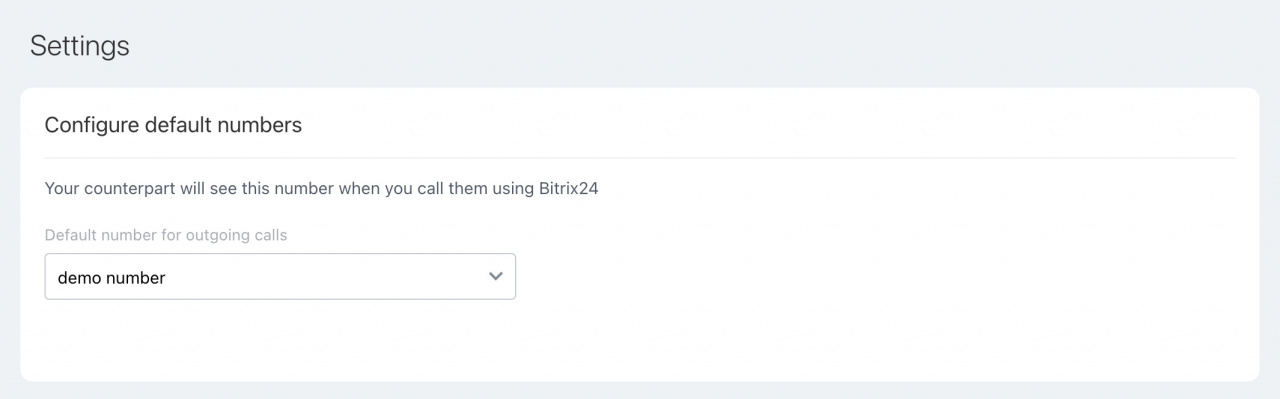The image presents a simple yet structured layout designed for configuring settings in a software application. The top left corner features the word "Settings" in bold black text. Surrounding the image, a greenish-gray border frames a central white background. Just beneath "Settings," also aligned to the top left, the heading "Configure Default Numbers" appears, also in bold black text.

Directly below this heading, a thin black line stretches horizontally across the image, providing visual separation. Beneath this line, a description reads: "Your counterpart will see this number when you call them using Bitrix24," rendered also in black text but without the boldness. The text to the right of this description remains empty.

Further down, in light gray text, the label "Default number for outgoing calls" is displayed. Below this label, a box contains the text "Demo Number" in bold black text. A downward arrow is situated to the far right within this box, indicating a dropdown menu. The entire area to the right and below this box remains empty, maintaining a clean and uncluttered appearance.

In summary, the image features the following elements in bold black text: "Settings," "Configure Default Numbers," and "Demo Number," all contributing to a user-friendly interface for configuring default numbers.